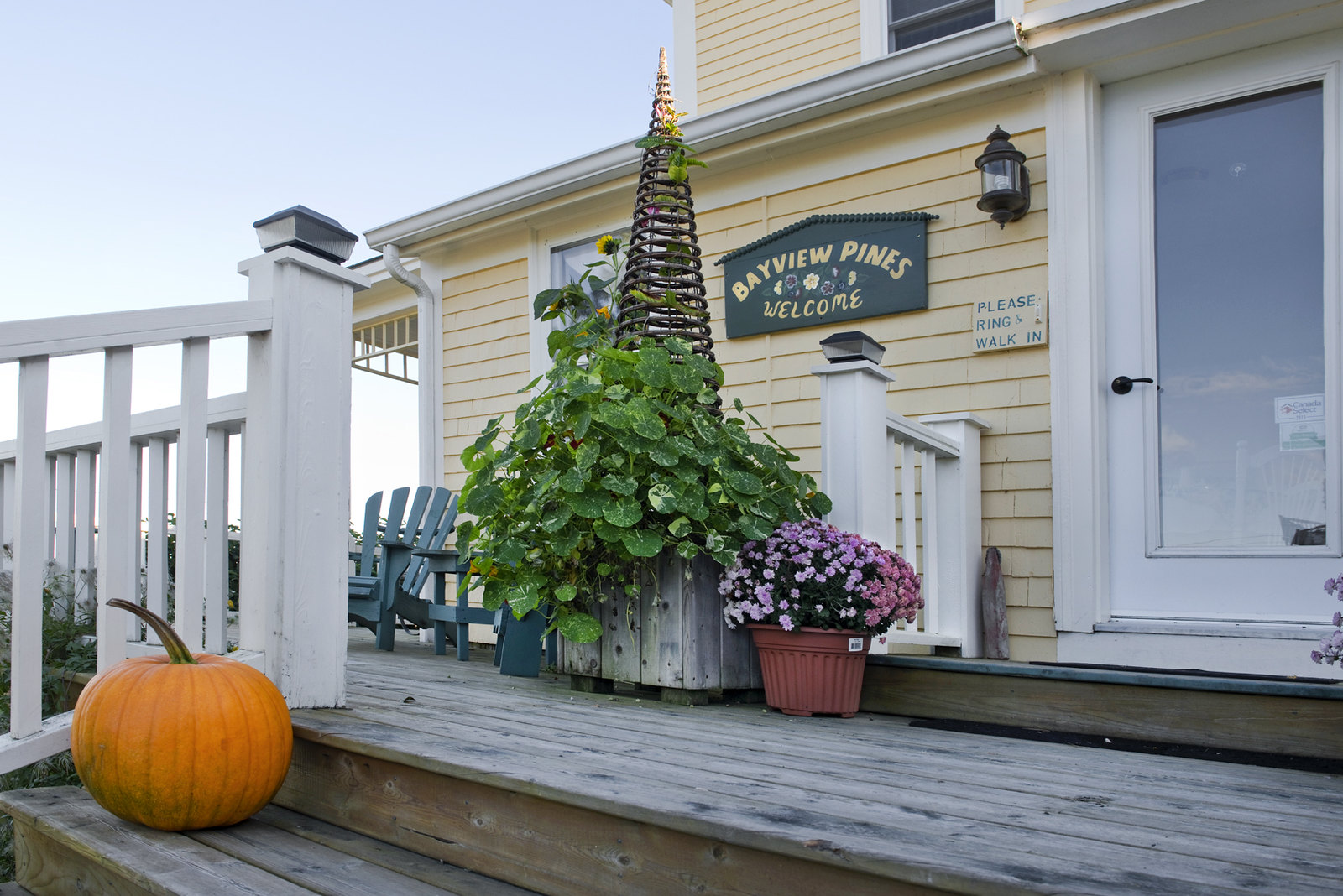The image depicts the front porch of a building with light yellow siding and a wooden deck. Prominent features include wooden stairs leading up to the deck, adorned with a large orange pumpkin. The porch is decorated with a green leafy plant in a wooden planter, along with a separate flower pot containing pink and purple flowers. There is a white fence and, to the right, a glass door with a white frame, beside which is a welcoming sign in green and yellow that reads "Bayview Pines, welcome." There's also a smaller sign instructing visitors to "please ring, walk in." Two green chairs are positioned on the deck, and the upper part of a second story is barely visible, bathed in a clear, light blue sky.